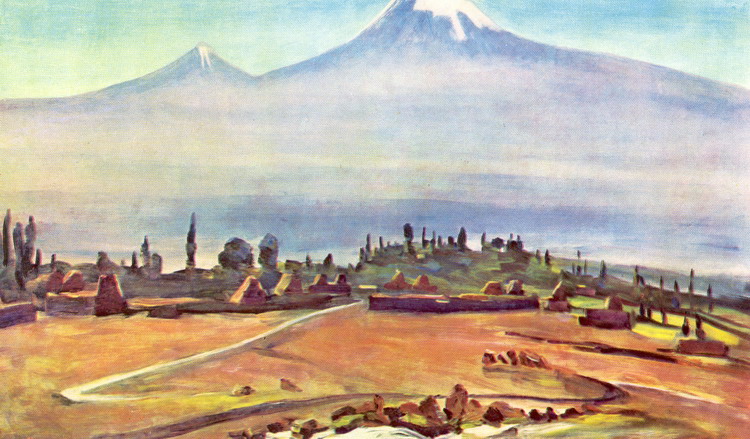This painting, titled "Byurakan" by Martiris Serrion, is a detailed landscape set within a horizontal rectangular frame. In the foreground, the bare land features a reddish-brown earth accentuated by rocks of various shapes. A path runs from the left, traversing the bottom of the painting. To the right of the path, vivid green grass grows towards the base of the scene, blending into the brown dirt. Scattered thin trees and possibly headstone-like shapes add texture to the mid-ground, interspersed with the structural forms of a city or cemetery.

Dominating the background is a grand, dark bluish-purple mountain with a snow-capped peak, standing tall and central within the composition. To its left, a smaller mountain rises, also featuring streaks of light blue and white. The mountains merge softly into the pale turquoise sky, creating a subtle blend where the boundaries of sky and mountain fade harmoniously. The overall scene is pastoral, outdoors, and well-lit, with distinct attention to the interplay of colors and softly blended forms, offering a tranquil yet complex portrayal of a contrasting natural and possibly human-influenced landscape.